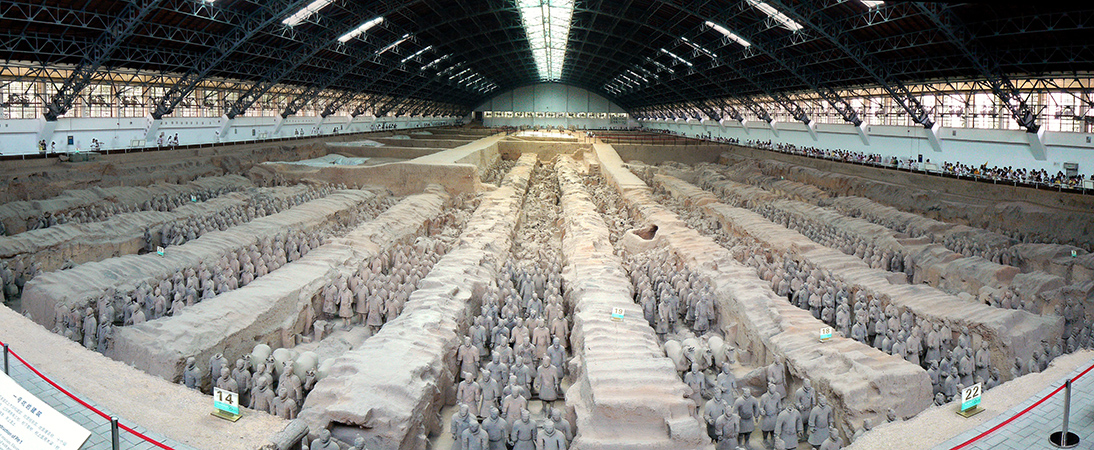The image captures an extensive museum exhibit, likely located in China or Korea, featuring a vast room with high, black or dark gray ceilings supported by metal framing. Suspended throughout the space, white lights illuminate the interior. The side walls of the room are blue, and beneath them, black iron pieces arch upwards towards the center, forming the ceiling structure. The back wall of the room is also blue with some unknown elements and white writing on it.

Dominating the exhibit are rows of meticulously sculpted figures, resembling soldiers, alongside horses, all crafted from stone and varying shades of gray to white. These figures are beautifully arranged between vertical barriers that resemble columns of brown clay or rock. The barriers run parallel across the exhibit space, creating numerous rows filled with the stone figures, adding to the grandeur of the scene.

On the left and right sides of the image, additional architectural features include white informational cards and red ropes attached to silver poles, roping off certain areas. Notably, there are signs posted on the barriers, evident from numbers such as 14, 18, 19, and 22 marking different sections of the exhibit.

Towards the bottom corners of the image, the floor appears to consist of blue tiles, with roped-off areas extending beyond the frame. The left side wall includes more numbers and signage similar to those seen on the barriers. The right side of the image shows a section with many actual visitors, indicating this is a popular and well-frequented exhibit within a large museum.

The combined details suggest that the exhibit likely depicts a "Terracotta Army" or a similar historical representation, drawing significant interest from visitors. The stunning scale and intricacy of the display make it a point of fascination, inspiring curiosity to learn more about its historical and cultural significance.